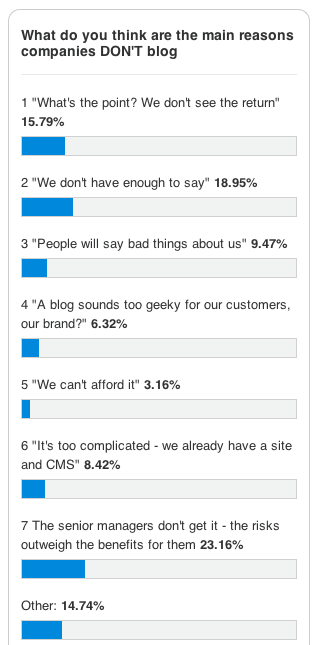This image displays a detailed statistics poll addressing the general question: "What do you think are the main reasons companies DON'T blog?" The word "DON'T" is notably emphasized in uppercase.

The poll presents eight distinct reasons, each with corresponding percentages of respondents who selected them:

1. "What's the point? We don't see the return" - 15.79%
2. "We don't have enough to say" - 18.95%
3. "People will say bad things about us" - 9.47%
4. "A blog sounds too geeky for our customers, our brand" - 6.32%
5. "We can't afford it" - 3.16%
6. "It's too complicated. We already have a site and CMS" - 8.42%
7. "The senior managers don't get it. The risks outweigh the benefits for them" - 23.16% (the highest response)
8. "Other" - 14.74%, representing any additional reasons companies may avoid blogging.

This comprehensive breakdown helps elucidate the diverse reservations companies have regarding the initiation of a blog.